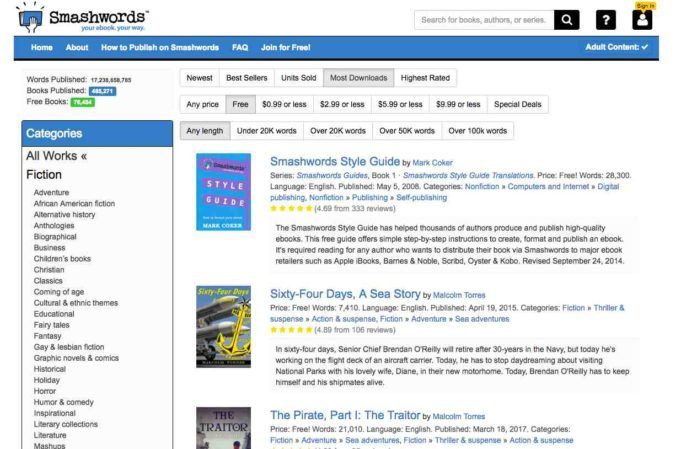The image showcases the Smashwords website interface. In the upper left corner, the Smashwords logo is prominently displayed with the tagline, "Your e-book, your way." On the right side, there's a search bar labeled "Search for books, authors, or series," accompanied by a question mark icon for assistance and a profile sign-in icon. Below this section is a blue navigation strip offering various options: from left to right, "Home," "About," "How to Publish on Smashwords," "FAQs," and "Join for Free." On the far right of this strip, there is an "Adult Content" checkbox.

A black horizontal line separates the navigation area from the main content below. On the left side, a section details the site's statistics, though slightly blurry: "Words Published: 17,238,858," "Books Published: around 413,271," and "Free Books: approximately 76,434."

Further down, the categories section lists a wide range of genres and topics available on Smashwords, including: "All Words," "Fiction," "Adventure," "African American Fiction," "Alternative History," "Anthologies," "Biographies," "Business," "Children's Books," "Christian," "Classics," "Coming of Age," "Culture and Ethics," "Themes," "Editorial," "Fairy Tales," "Fantasy," "Gay and Lesbian Fiction," "Graphic Novels and Comics," "Historical," "Holiday," "Horror," "Humor and Comedy," "Inspirational," "Library Collections," "Literature," and "Mashups."